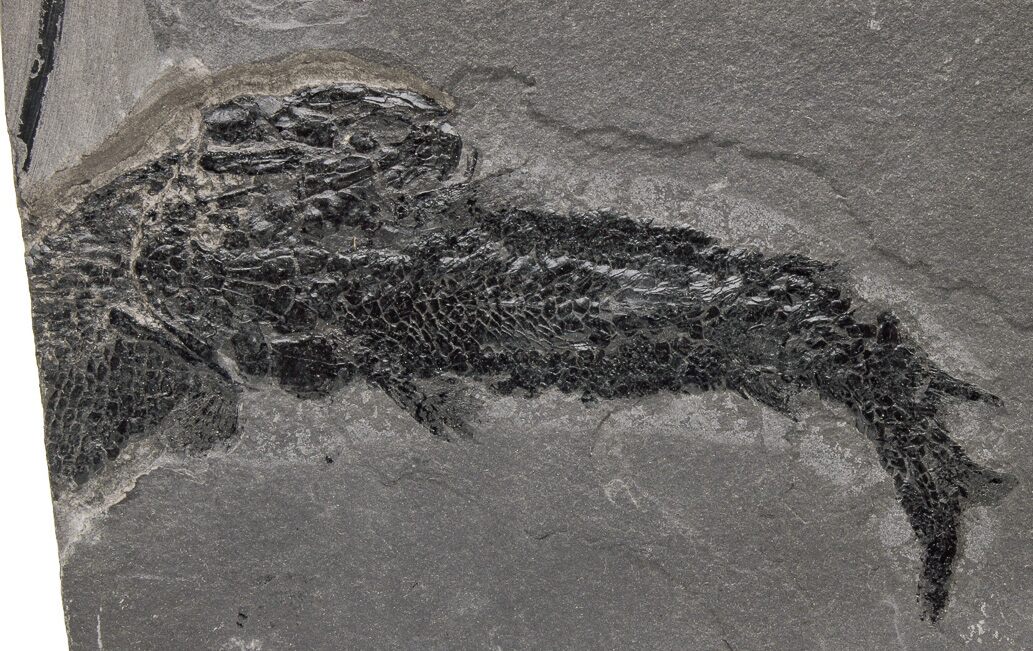The image depicts a fossil embedded in a gray, sandy-textured stone. The fossil itself is markedly darker, ranging from deep black to dark gray. Centered in the stone, the fossil displays a distinct face that resembles that of a squirrel or chipmunk, with a visible eye on the right-hand side and a nose. Beneath the face, the body extends downward, ending in a fin-like shape towards the bottom right, hinting at a sea creature-like appearance with scaly textures reminiscent of a fish's tail. The stone around the fossil shows multiple cracks and lines, particularly above the fossil, suggesting its age and fragility. The overall lighting of the image is dim, emphasizing the fossil's dark shading against the gray rock background.